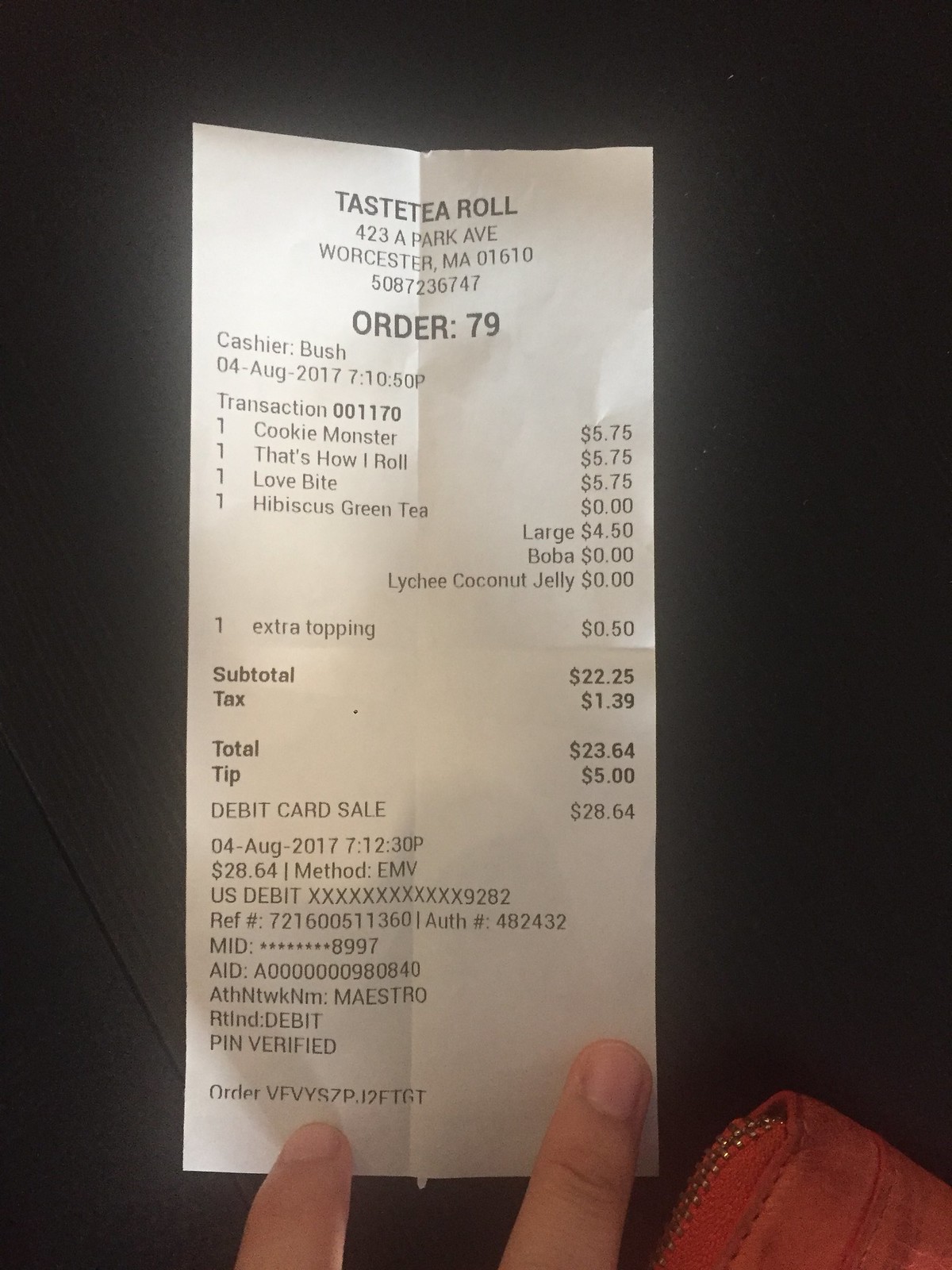The photograph showcases a white receipt from Tasty Roll, positioned against a black background. The receipt details an order from 423A Park Avenue, Worcester, Massachusetts, 01610, and includes the establishment's phone number. The order, number 79, was processed by Cashier Bush. 

Detailed information on the transaction includes the date, August 4, 2017, and it shows that items ordered were Cookie Monster for $5.75, That's How I Roll for $5.75, Love Bite priced at $0.00, Hibiscus Green Tea also at $0.00 with additional charges for a large size at $4.50, boba for $0.00, lemon lychee coconut jelly for $0.00, and an extra topping for $0.50. The subtotal amounts to $22.25, with a tax of $1.39 resulting in a total of $23.64, plus a $5.00 tip, bringing the debit card transaction to $28.64.

The image reveals two light-complexioned fingers holding the receipt from the bottom. In the lower right corner of the photo, part of a piece of clothing or a purse is visible.